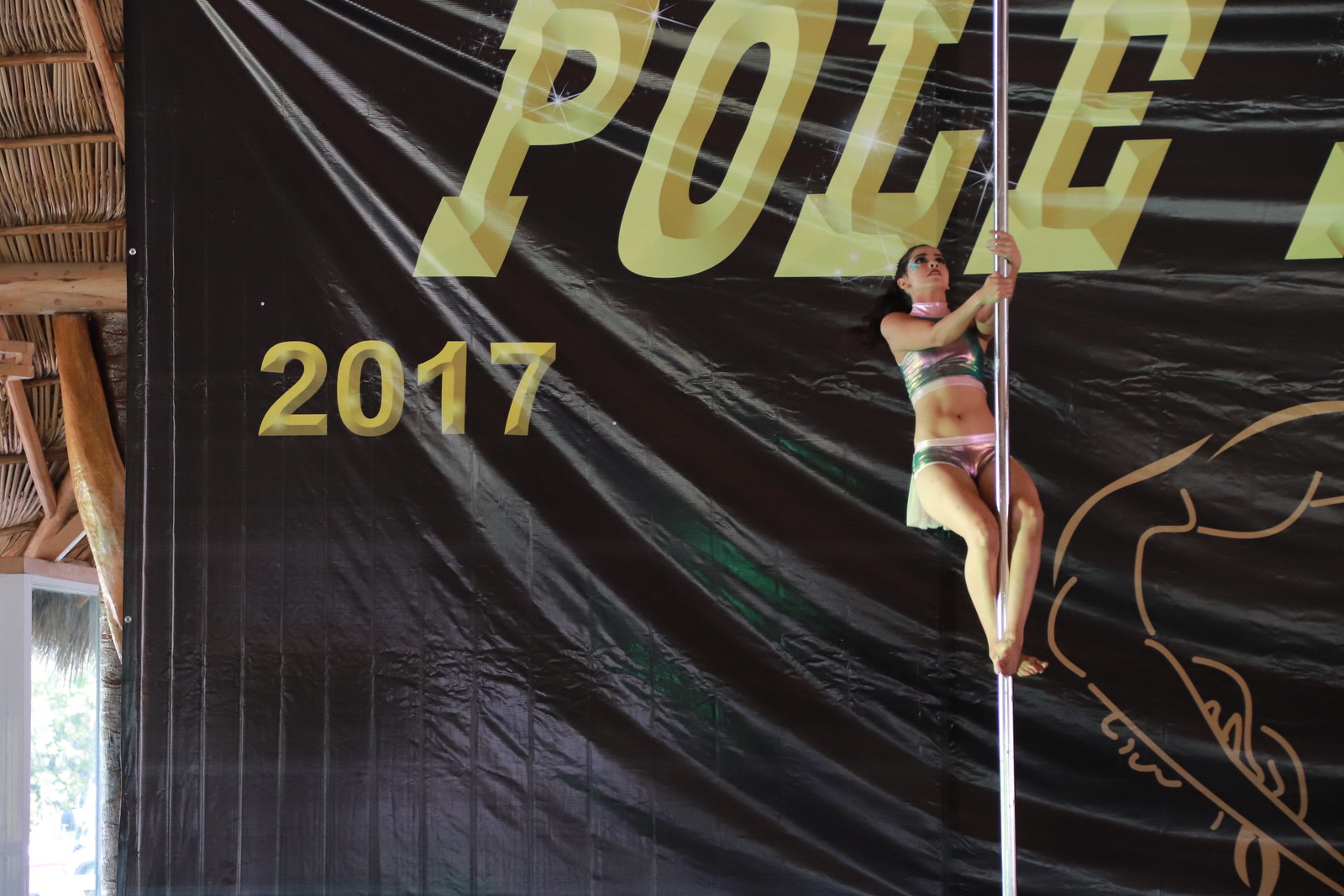The image captures a vivid moment at a pole dancing competition. Dominating the right half of the photograph, a Caucasian woman with dark brown hair and light skin is intricately wrapped around a silver-toned pole. Her attire consists of a glittery green tube top and shorts, both dazzling under the light illuminating her from the left. She displays an athletic physique, with muscular midriff exposed. Her hands firmly grasp the pole while her legs are entwined around it at the ankles, showcasing her flexibility and strength. 

Behind her, a large black tarp serves as a backdrop, prominently featuring the word "POLE" in embossed yellow letters at the top and the year "2017" situated more to the left. The tarp shows signs of wear, sagging and wrinkling towards the center. On the extreme right edge, a fragment of another letter is barely visible, hinting at an extended word or logo beyond the frame. Adding to the scene's exotic ambiance, the left side of the image reveals a straw-like thatched ceiling supported by wooden beams, with sunlight streaming through a window below, creating a dynamic interplay of light and shadow around the performer. The woman gazes upwards, her facial features partly obscured, contributing to the air of focused determination.